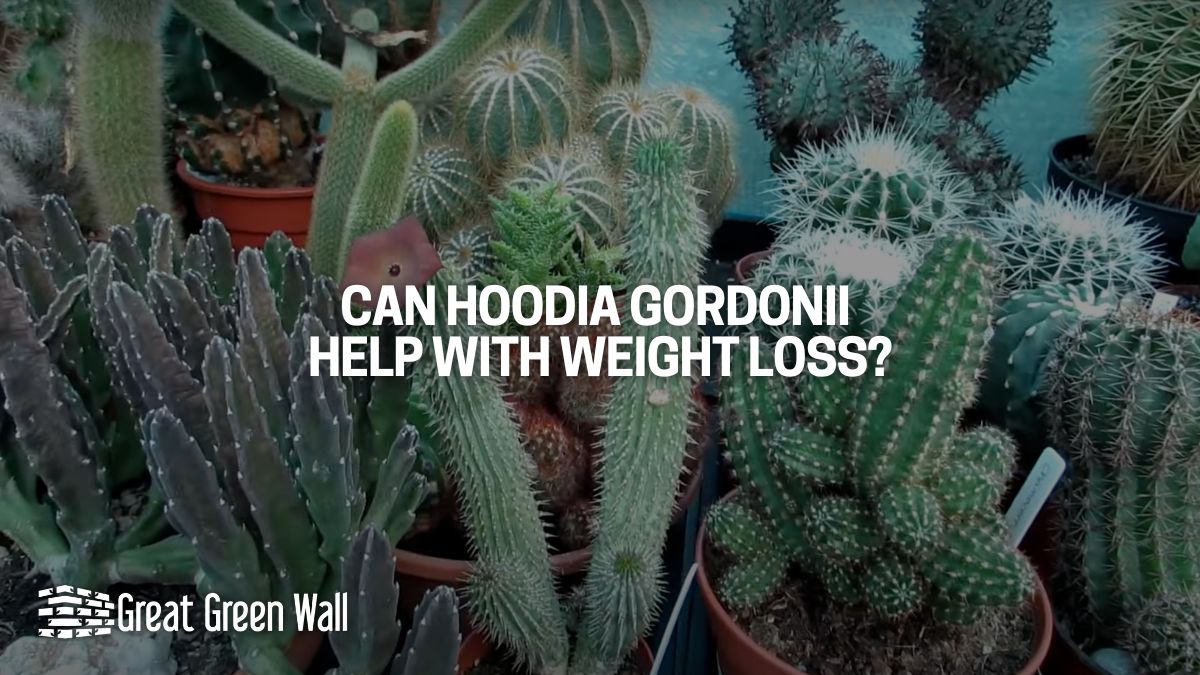The image is a color photograph featuring a variety of potted cactuses set against a turquoise background. The cactuses, which are of different types and shapes— including long and tall, football-shaped, and round varieties— are housed in various pots made of materials like terracotta, ceramic, and plastic. There are at least eleven distinct types of cactuses visible. The cactuses are evenly spread throughout the image, while the center is overlaid with white, all-capital text that reads, "CAN HOODIA GORDONII HELP WITH WEIGHT LOSS?" In the bottom left corner, there is a white brick wall logo accompanied by the text "GREAT GREEN WALL." The overall setting suggests that this image might be an advertisement for a weight-loss product involving cactuses. The colors in the image include light blue, green, white, orange, brown, tan, and gray.